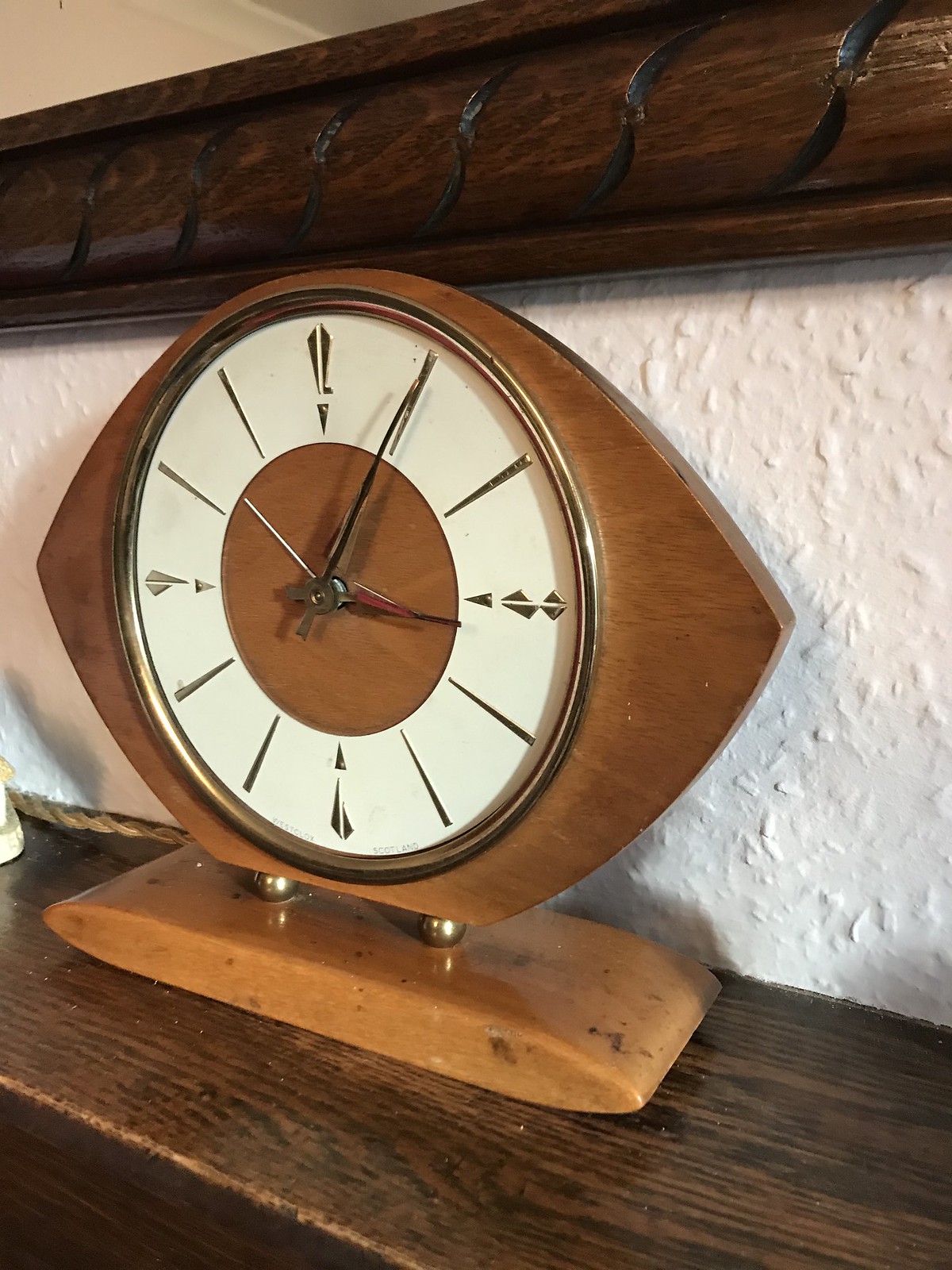This photograph captures a detailed and intriguing mantel clock situated on a dark wooden mantel inside a house. The clock, which exudes an antique charm, is presented on a diagonal wood shelf that extends from the bottom right to the middle left of the picture. Crafted in an eye-shaped wooden frame with a slightly flattened bottom, the clock rests on an oblong light-colored wooden base, complete with two circular balls at its center. The clock face features an off-white background with a central brown circle, encased in a gold bezel. The time displayed is 3:05, with stylized black hands. Notably, the hour positions are marked by simple vertical lines, except for the 12, 3, 6, and 9 o'clock positions, which are highlighted by more elaborate lines. Enhancing the composition, an ornate wooden molding with an S-shaped design is visible above the clock, while the backdrop consists of a textured white wall, adding depth and character to the setting. The photograph's diagonal perspective further accentuates the clock's elegant and unique design.